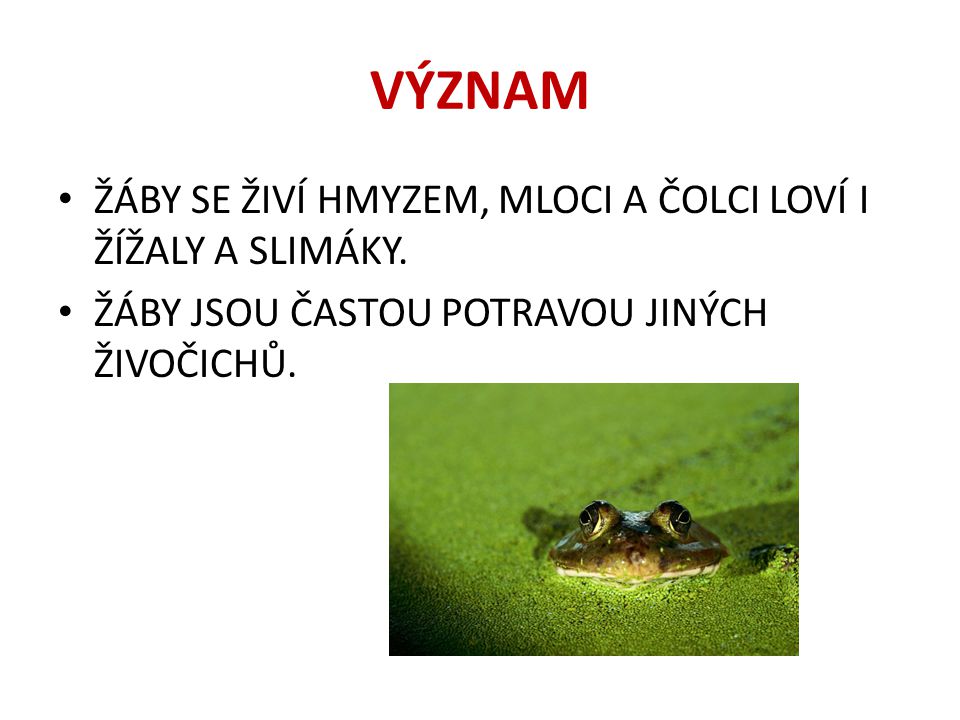The image depicts a PowerPoint slide that appears to be for an educational presentation, possibly for a high school or college course, written in an Eastern European language. The slide has a white background with a title at the top in large, red, all-caps sans-serif text that reads "VIZNAM." Below the title are two bullet points, written in black all-caps sans-serif text, containing a series of words with various diacritics. The first bullet point includes "Zabi, C, Zivi, Haimazem, Melokai, A, Kolchi, Lovi, I, Zazali, A, Slemaki," while the second reads "Zabi, Zu, Kastu, Portavu, Jianch, Zivakuchu."

Situated in the bottom right corner of the slide is a smaller photograph of a green bullfrog partially submerged in a pond with only its head and eyes visible above the densely packed algae-covered water. The algae gives the surface of the pond a light green color, which fades to black towards the lower left corner of the photograph. The frog's eyes are black, creating a contrast against its green and yellowish body. The overall style and layout of the slide suggest it is designed for a formal presentation, potentially discussing a topic related to frogs.